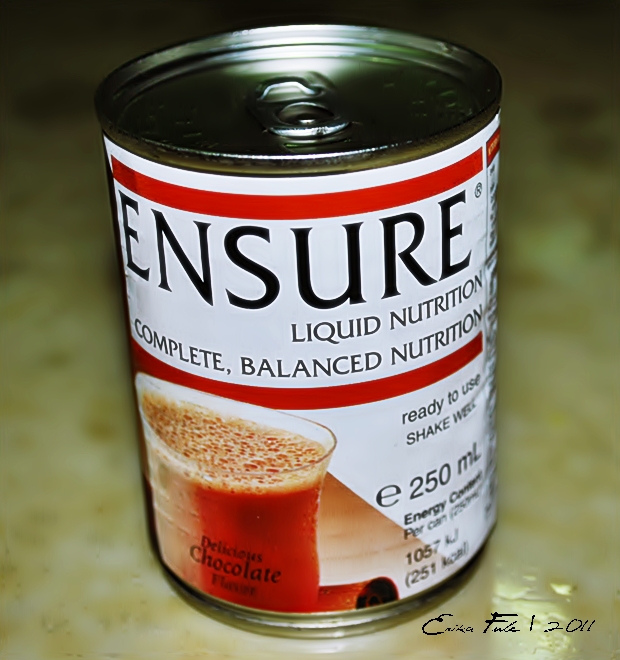This color photograph portrays a digitally manipulated image of a cylindrical can of Ensure Liquid Nutrition prominently centered against a blurry marble-like background that resembles liquid. The can, which appears to be an older version, features a white label with a red stripe at the top. "Ensure" is written in large black capital letters, followed by the phrases "Liquid Nutrition" and "Complete Balanced Nutrition" in smaller type. On the left side of the label, the flavor is specified as "Chocolate," accompanied by an image of a transparent cup filled with a brown liquid. This cup is labeled "Delicious Chocolate Flavor" in black letters, with visible bubbles on top. Additional details include metrics in milliliters and kilocalories on the left. The can has a metallic pull-tab top, highlighted by lighting. In the lower right-hand corner of the image is a signature in thin black ink reading "Erica Foula" followed by the number "12011," suggesting the image might be part of a numbered art series. The edges of the image appear cut out and pasted onto the unique background, enhancing its artistic appeal.